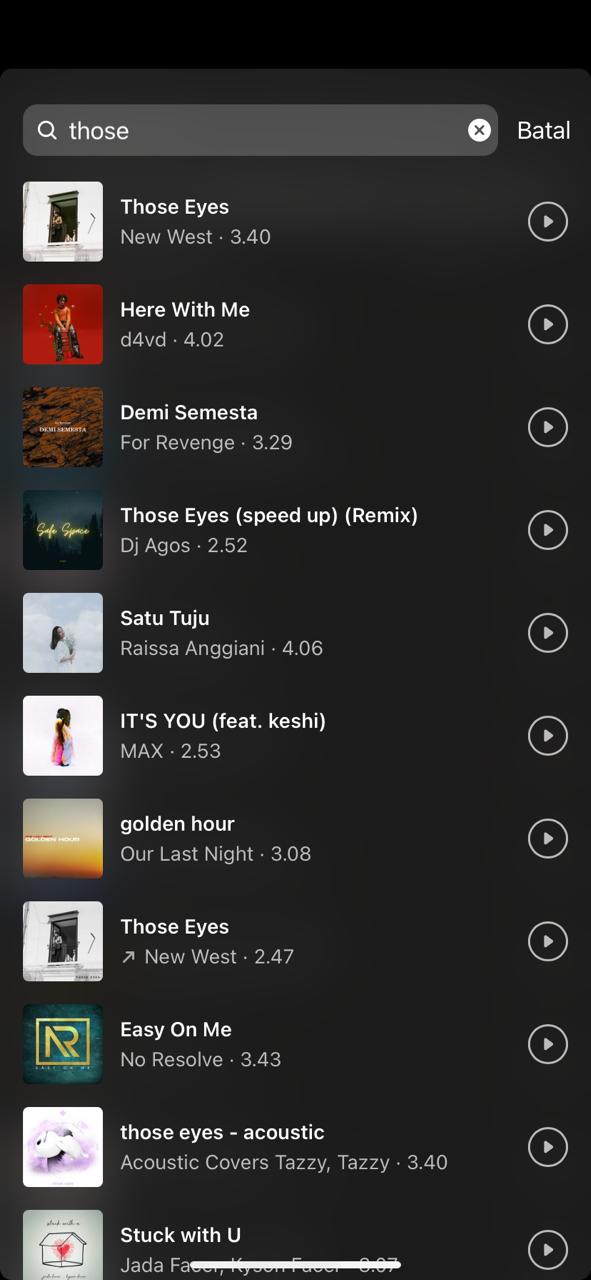The image features a black background showcasing a music playlist interface. At the top, there is a search bar containing the text "those eyes" with a small 'X' icon next to it for clearing the search. Each song on the list has a circular play button icon on its right side. The following tracks are displayed, each with their respective durations:

1. "Those Eyes" by Newest – 3 minutes, 40 seconds
2. "Here With Me" by D4vd – 4 minutes, 2 seconds
3. "To Me" by Semester for Revenge – 3 minutes, 29 seconds
4. "Those Eyes (Sped Up Remix)" by DJ A – 2 minutes, 52 seconds
5. "2 To 2 You" by Restaurant NASA – 4 minutes, 6 seconds
6. "It's You (featuring Keshi)" by MAX – 2 minutes, 53 seconds
7. "Golden Hour" by Our Last Night – 3 minutes, 8 seconds
8. "Those Eyes" by New West – 2 minutes, 47 seconds
9. "Easy On Me" by No Resolve – 3 minutes, 43 seconds
10. "Those Eyes (Acoustic Cover)" by Tazzy Tazzy – 3 minutes, 40 seconds
11. "Stuck With You" – partially shown at the bottom, with the duration cut off due to the interface limits.

The list appears to be a curated phone playlist, implying it was not generated by any specific music program.